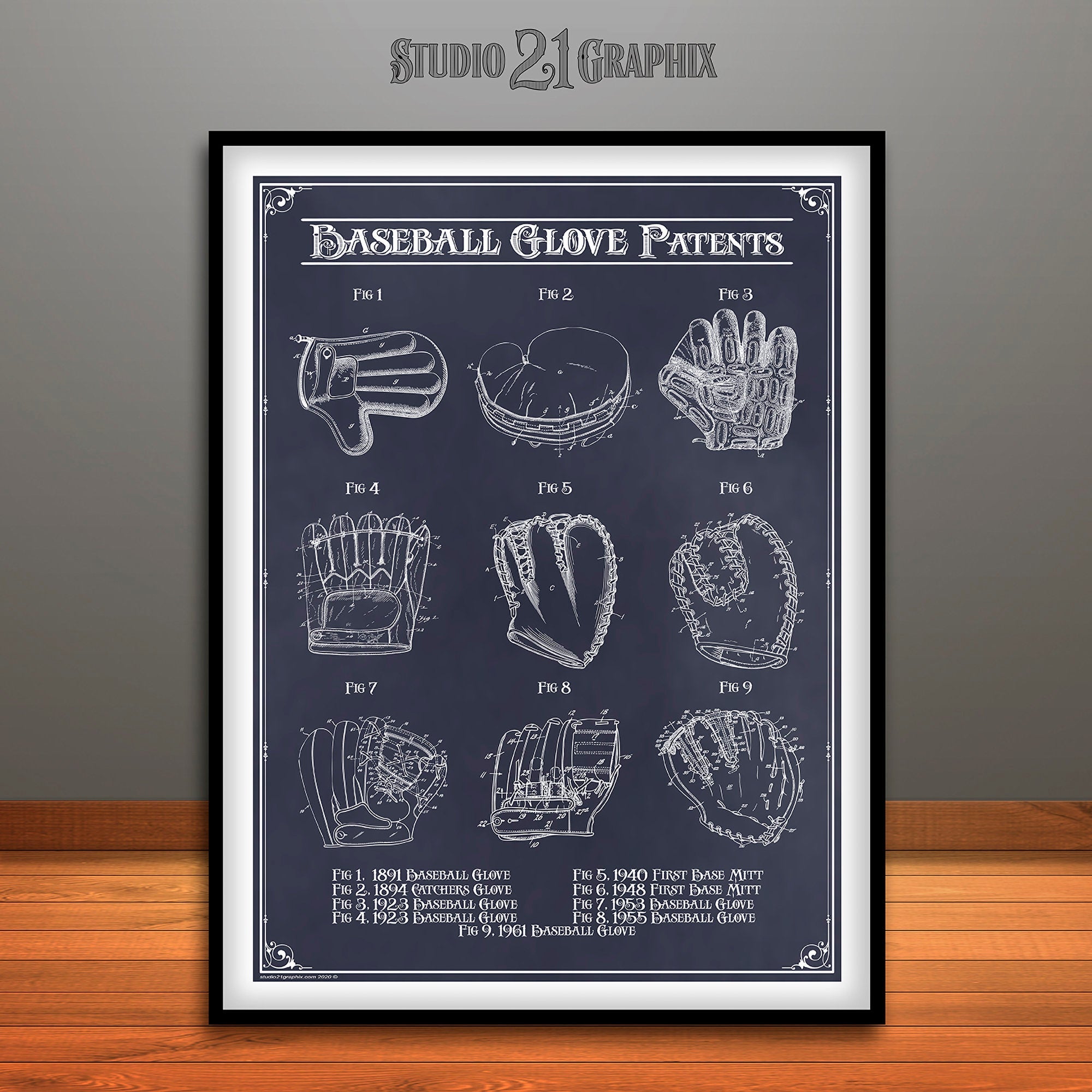In this image, there is a detailed poster showcasing the evolution of baseball glove patents. The poster is encased in a silver-white frame with an outer black border and positioned against a wall. At the top, the poster prominently features the title "Baseball Glove Patents" in capital letters. Surrounding the poster's gray background, there are nine detailed white drawings of various baseball gloves, each marked as a figure accompanied by a year and description. The figures are labeled as follows: Figure 1 is an 1891 Baseball Glove, Figure 2 is an 1894 Catcher's Glove, Figure 3 is a 1923 Baseball Glove, Figure 4 is another 1923 Baseball Glove, Figure 5 is a 1940 First Base Mitt, Figure 6 is a 1948 First Base Mitt, Figure 7 is a 1953 Baseball Glove, Figure 8 is a 1955 Baseball Glove, and Figure 9 is a 1961 Baseball Glove. Above the framed poster, the wall features the inscription "Studio 21 Graphics." The wall behind the frame is a gradient gray, transitioning from dark gray at the bottom to a lighter shade further up. The frame itself is sitting on a surface that resembles orange-toned hardwood.